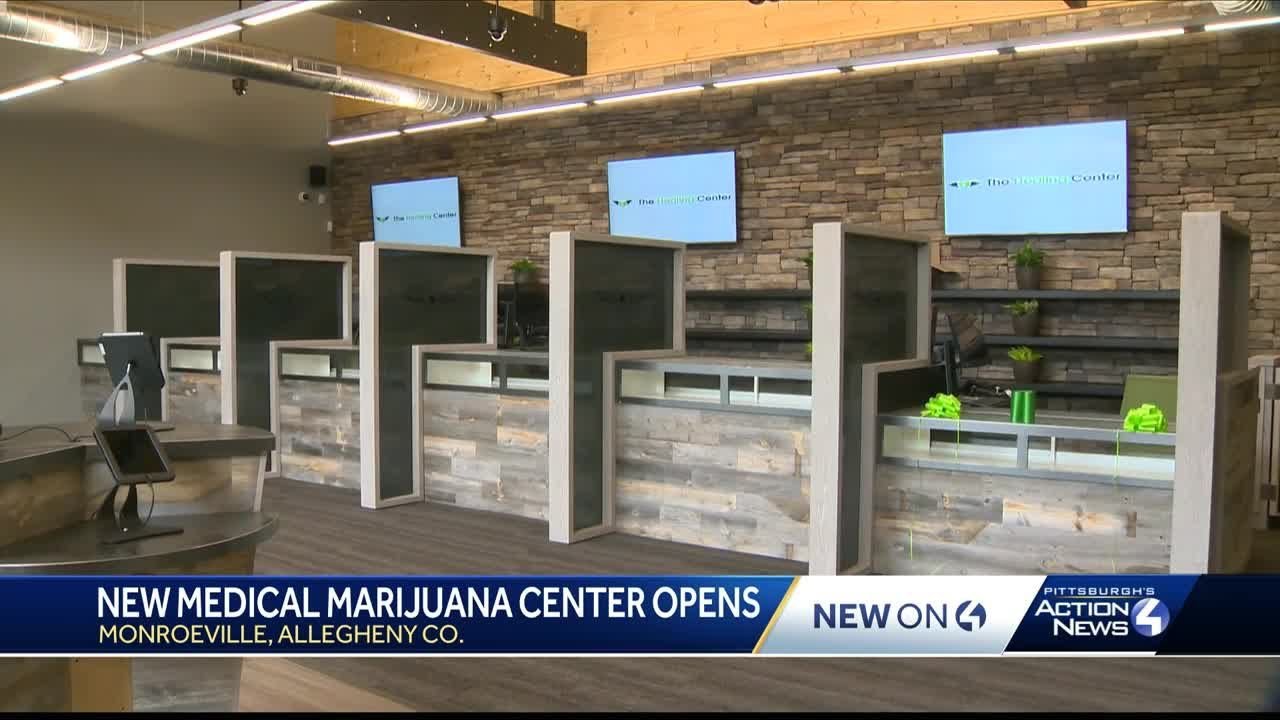This image is a still from a news broadcast detailing the recent opening of a new medical marijuana center in Monroeville, Allegheny County, as indicated by the blue and white text banner at the bottom of the screen which reads "New Medical Marijuana Center Opens, Monroeville, Allegheny County, New on 4, Pittsburgh's Action News." The interior depicted in the photograph features a spacious, industrial-style room with high, open ceilings that reveal support beams and exposed tubing. The back wall is constructed of off-white, tan, or light teak brick, against which three large flat-screen monitors are mounted. There are five counters or desks aligned in a row, separated by wooden dividers that resemble a bank's teller stations. These desks have fronts made of grayish-brown planks and the counter on the right-hand side holds two bundles of green objects alongside two dark green cylinders. The entire setting is brightly lit by fluorescent lights, giving a clear view of the industrial yet welcoming atmosphere of the center.